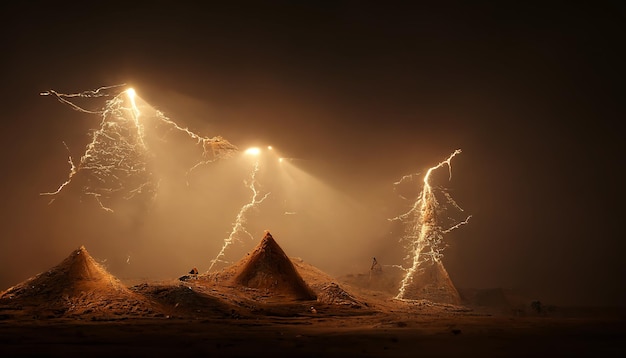The image depicts an eerie nighttime scene featuring sharp, pyramid-like mounds, possibly resembling hills or tents, in hues of orange and red. These mounds are accentuated by three distinct lightning bolts streaking from a dark, black sky. The lightning bolts, with branches similar to a river's tributaries, illuminate the scene, creating a stark contrast between the bright strikes and the shadowy foreground. The lightning predominantly strikes between and around the mounds, casting an almost otherworldly glow that highlights their sharp peaks. The surrounding area is dim and shadowy, adding to the unsettling and almost frightening atmosphere of this graphic depiction. The interplay of the lightning with the dark and the illuminated mounds creates a captivating and dramatic visual effect.